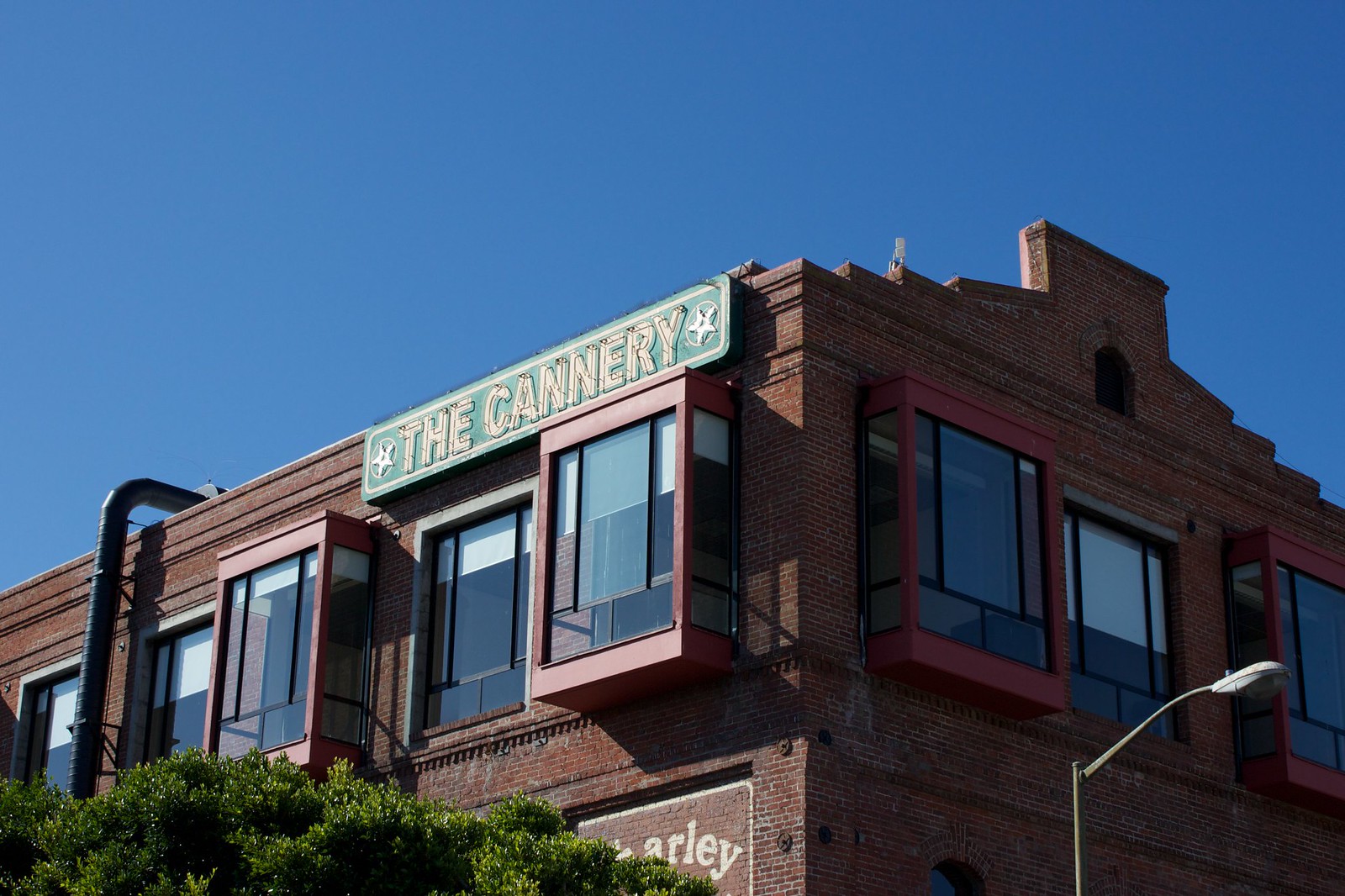The image captures a detailed street-level view looking up at the corner of a large, red brick building. The building appears to be two or three stories tall and could be an old factory renovated into housing. Dominating the top of the building is a neon sign that reads "The Cannery," flanked by small white stars on either side. Every other window on the top floor features a distinct red extrusion, adding architectural interest and possibly indicating bench seating at the bottom inside. The clear blue sky serves as a serene backdrop, entirely free from clouds. The bottom right-hand side of the picture features a streetlamp, while the bottom left reveals the tops of some green bushes and trees, adding a touch of nature to the urban setting.